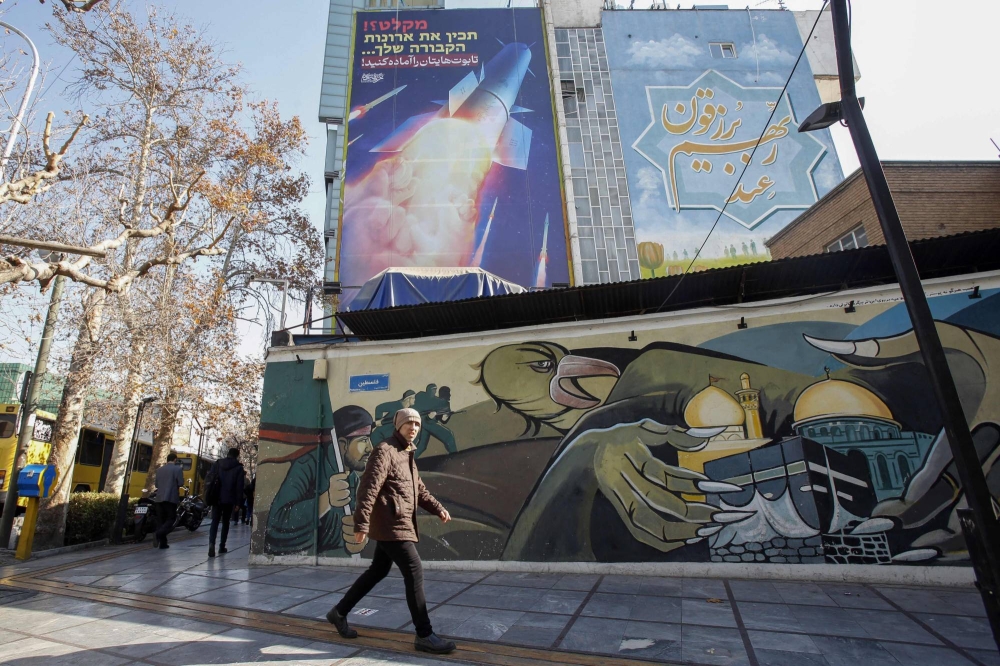In this vibrant daytime street scene, a man strides confidently in the foreground, his face illuminated by sunlight as he looks directly at the camera. He is dressed in a brown jacket, black pants, and a cap. Behind him, an intriguing mural adorns a large building, portraying a yellowish eagle with sharp talons clutching a cartoon mosque, while people with guns and a flag are depicted to the left. Further back, another mural illustrates a rocket taking off, featuring blue hues and possibly Arabic or Jewish script. The busy street includes trees to the left, a utility pole on the right, and another person in the background walking away. The sidewalk beneath the man has a glossy grid pattern, and vehicles can be seen in the distant background.